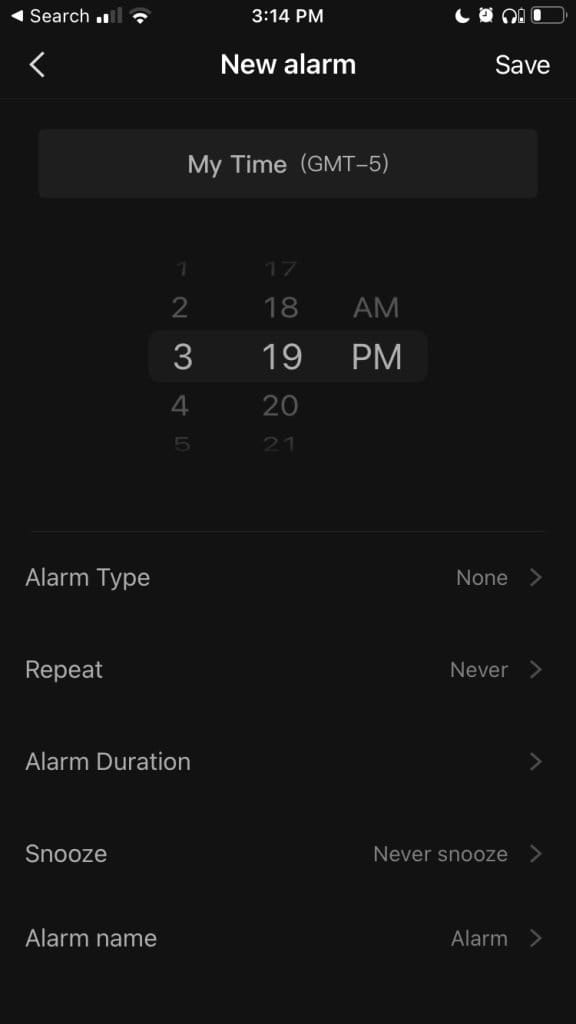The image is a screenshot of a mobile phone displaying the interface for setting a new alarm in dark mode. The status bar at the top shows standard icons: a backwards play button labeled "search," two bars of cellular signal, a weak Wi-Fi connection, the current time "3:14 PM," and a moon icon indicating dark mode is active. Additionally, there is an icon showing that headphones are plugged in and a battery icon that suggests a low battery level.

In the main section of the screen, the user is in the process of creating a new alarm. The current time zone is displayed, and they are setting the alarm for "3:19 PM," just five minutes ahead of the current time shown at the top of the phone. The "Save" button is located in the top right corner. Below the time setting, various customization options are listed, including alarm type, repeat schedule, alarm duration, snooze, and alarm name.